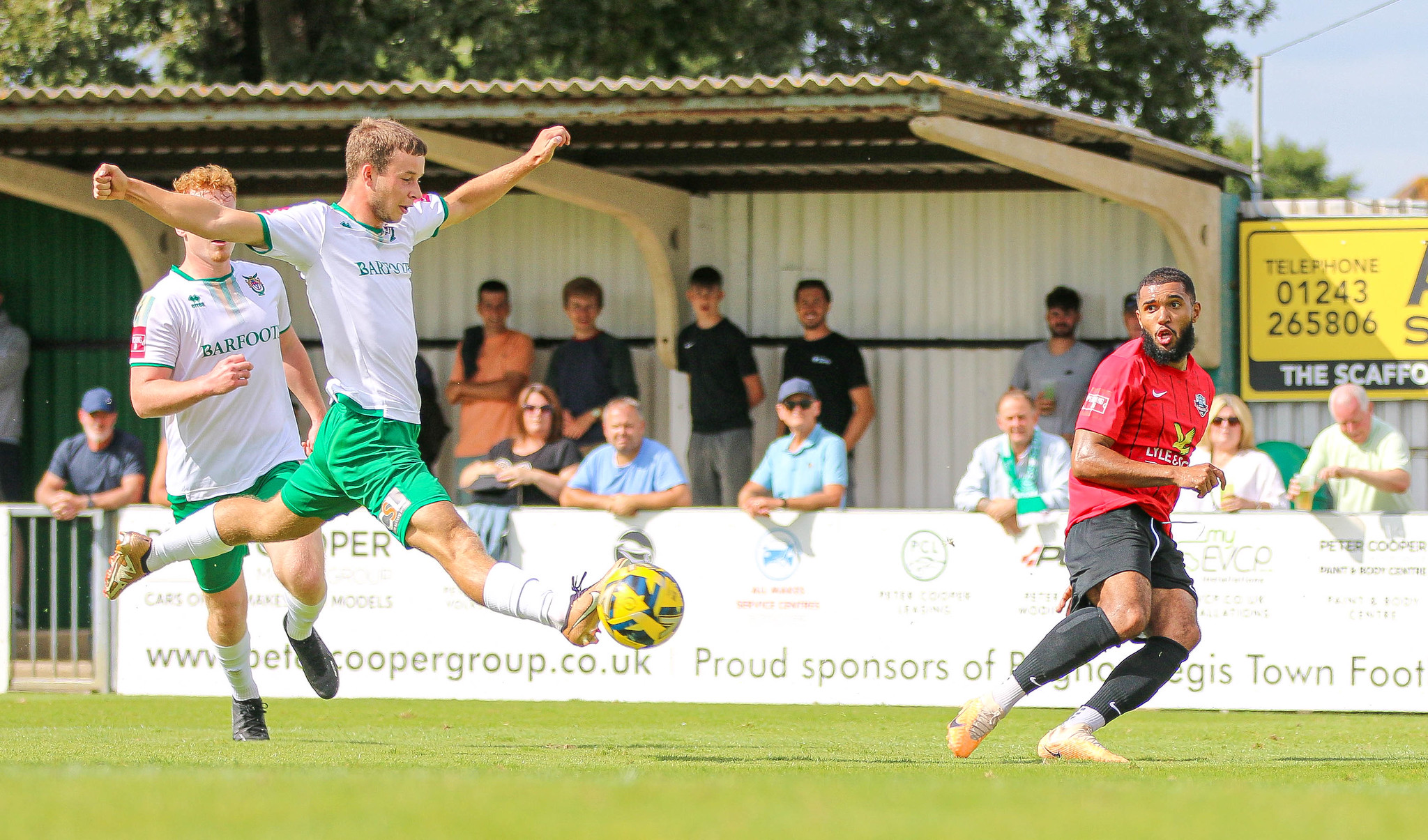In this vibrant outdoor soccer match scene set against a clear blue sky and lush green trees, action unfolds on a pristine, bright green grass field surrounded by a white fence. Enthusiastic fans lean against the fence, watching intently. Central in the foreground, a young player in a dynamic mid-air pose, wearing a white jersey with "barfoot" on it and green shorts, prepares to kick a bright yellow soccer ball. His white, high socks and athletic form are clearly visible as he splits the air. Snapping into focus behind him, a teammate in a matching white jersey and green shorts charges forward, contributing to the intense moment. Opposing them is a player in a red Nike jersey, black shorts, and high black socks with Nike logos, his eyes fixed on the scene as he dashes forward, face marked by a distinct beard. The field is emblazoned with a prominent yellow billboard in the background, displaying "betcoopergroup.co.uk" and a phone number, signaling proud team sponsorship. The sunny, clear day and meticulous details capture the passionate energy and camaraderie of this lively soccer match.